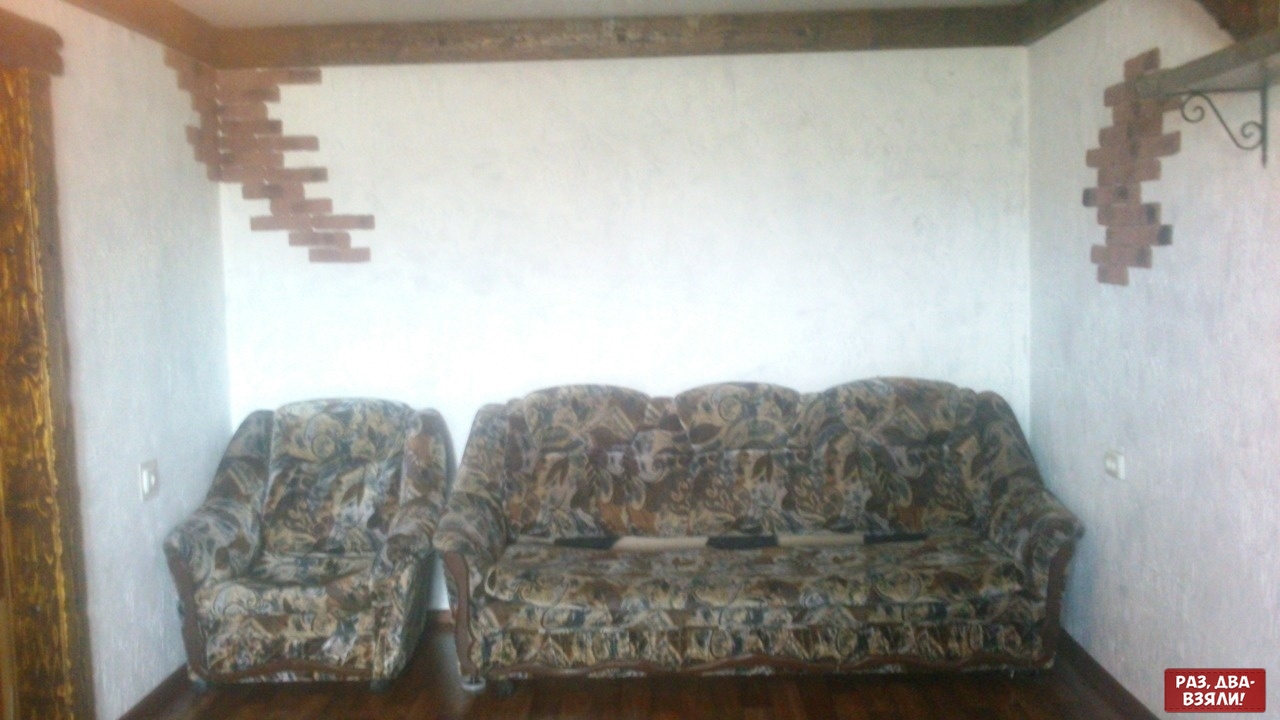The image depicts a cozy living room furnished with a matching couch and chair, both featuring an intricate, multi-colored fabric pattern dominated by shades of brown, grey, and orange. The seating set is arranged against a white wall, which is accented by wood trimming at the top, giving the room a warm, homey feel. The wall behind the couch has a unique decor with red brick accents that rise upward to the left, resembling a stairwell design, and additional brick adornments on the right, separated by a visible wooden beam supporting the ceiling.

To the left of the image, a light to dark brown wooden door frame is visible, along with two cream-colored light switches located just above the armrest of the chair and couch respectively. On the far right, there's a dark grey shelf held up by a metal bracket. At the bottom right corner of the image, a red square sign with white text reading "PA3 ABA B3R" and an upside-down triangle with an "N" can be seen. The floor, partially visible, is a dark brown hardwood, adding richness to the room's aesthetic.